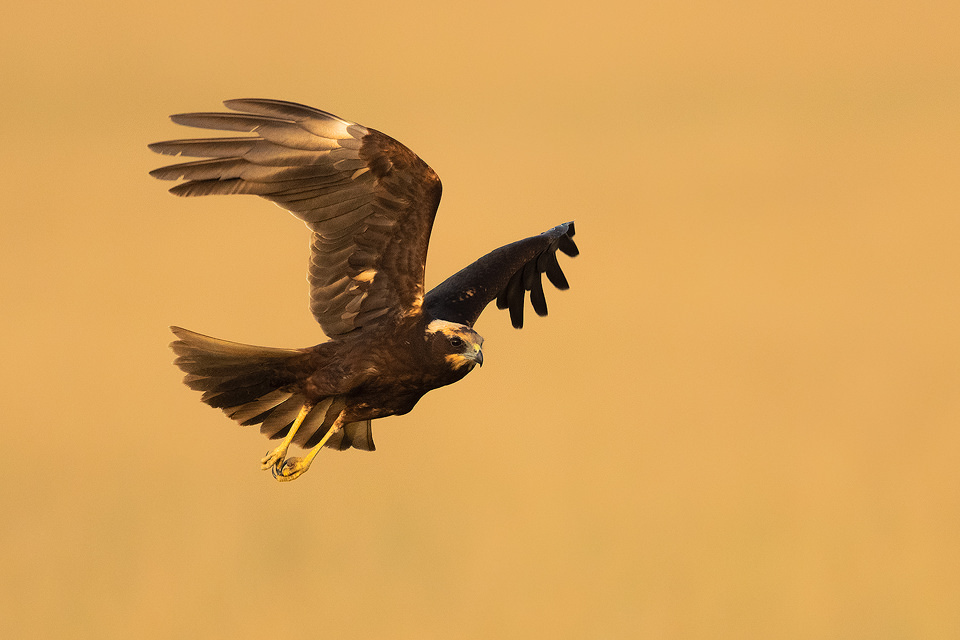This is a close-up, computer-generated image of a large hawk flying against a solid, hazy orange-gold background that resembles a dust storm. The bird is depicted in mid-flight, heading towards the right side of the image, with its wings stretched upward mid-flap. The hawk's feathers exhibit a range of brown shades, with lighter, yellowish tips, and the wings feature darker shadowed areas. Its body and tail feathers are primarily brown, fanning out behind it. The bird's white face is complemented by yellow cheeks and small, dark brown eyes. The beak is short, black-tipped with a hint of yellow at the base. Its yellow legs and talons are hanging underneath, clenched and visible. The background is devoid of any other elements, ensuring the focus remains on the majestic bird of prey soaring through the sky.